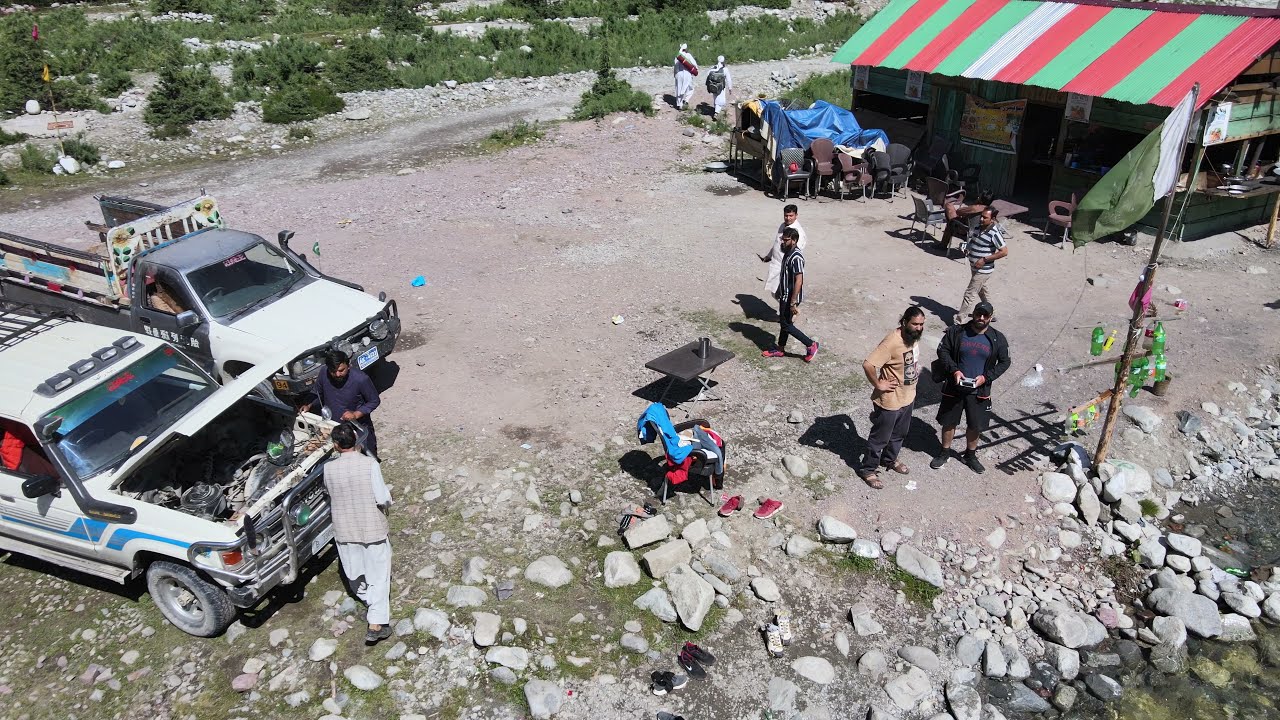This landscape-oriented, drone photograph offers a detailed aerial view of a barren, rocky outdoor scene, likely situated in a third-world country, under midday lighting. In the bottom left corner, the image captures two parked vehicles. One vehicle has its hood popped open, with two men inspecting the engine; the man on the left sports a beige long-sleeve shirt with black pants and sandals, while his companion wears an all-black outfit with a ball cap. Adjacent to these vehicles is a truck with a flatbed trailer, parallelly parked.

To the right side of the image, a windsock on a pole stands out, with two men nearby looking towards it—one dressed in a beige long-sleeve shirt and black pants, and another in all-black attire with a ball cap. Scattered across the rocky foreground are several additional people, some of whom gaze up at the camera.

The upper right part of the image features a tented structure with a distinct roof striped in red, green, and white, made from corrugated metal or sheet metal. A blue tarp is positioned in front of this structure, covering some stacked furniture. Further behind this setup, two men in long white garments walk along a gravel road.

The earthy tones of the rocky ground, interspersed with occasional bushes, provide a stark contrast to the vibrant colors of the tents and tarps, contributing to the realism of the photographic representation.